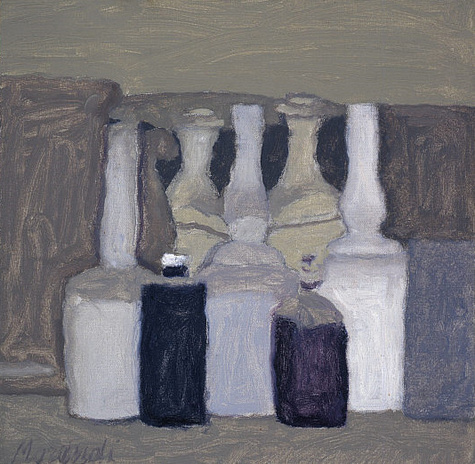This image is a hand-done piece that uses either watercolor or chalk pastel applied to a heavy stock, tan paper. The painting is square and exhibits a mix of implied and detailed style. It features a series of bottles filled with various fluids. In the background, there are five taller bottles, while the foreground is occupied by three shorter bottles. The bottles are outlined in black or dark colors, with white lids, and are highlighted in a variety of light shades, including gray, white, and blue. The top, bottom, and sides of the image contain shades of gray and hints of blue. Two black squares are positioned in the middle, flanking three white structures with two gray ones in between. The artist's signature is located in the left-hand corner and appears to be from someone whose name begins with "M-A-R" or "M-A-Z-A-N-D-A." Touches of blue, white, yellow, and black enhance the overall aesthetic of the artwork, which exudes a refined, yet somewhat abstract quality.